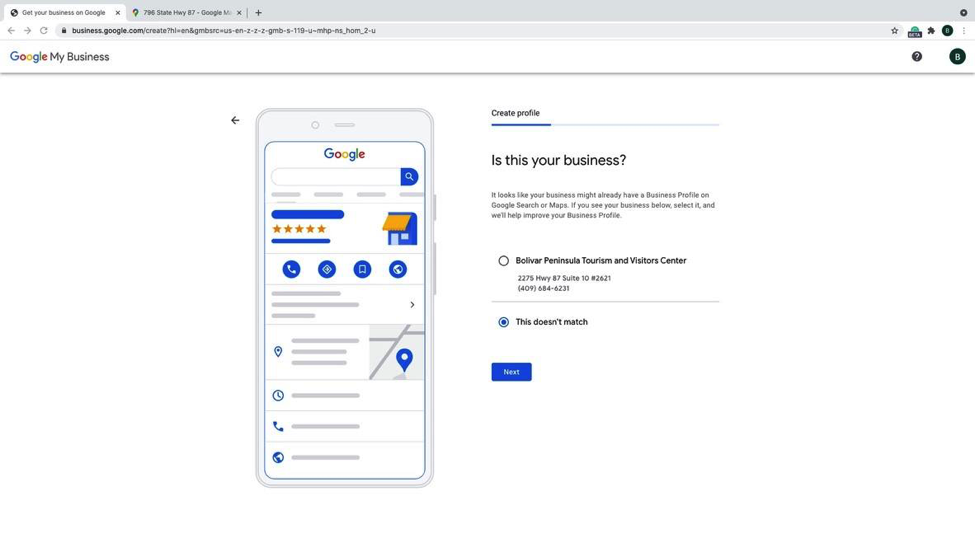This image depicts a web browser with two open tabs. The highlighted tab is titled "Get Your Business on Google," and the web address displayed is "business.google.com." In the white bar that spans the bottom of the browser window, the text reads "Google My Business." The user profile is represented by a green circle containing a white "B."

The main section of the window features an image of a cellphone positioned to the left. To the right of this image, the text "Create Your Profile" is displayed prominently. Beneath this, in black font, appears the question "Is this your business?" followed by a short paragraph consisting of three lines. Further down, there are two options available for selection, with the option "This doesn't match" currently chosen.